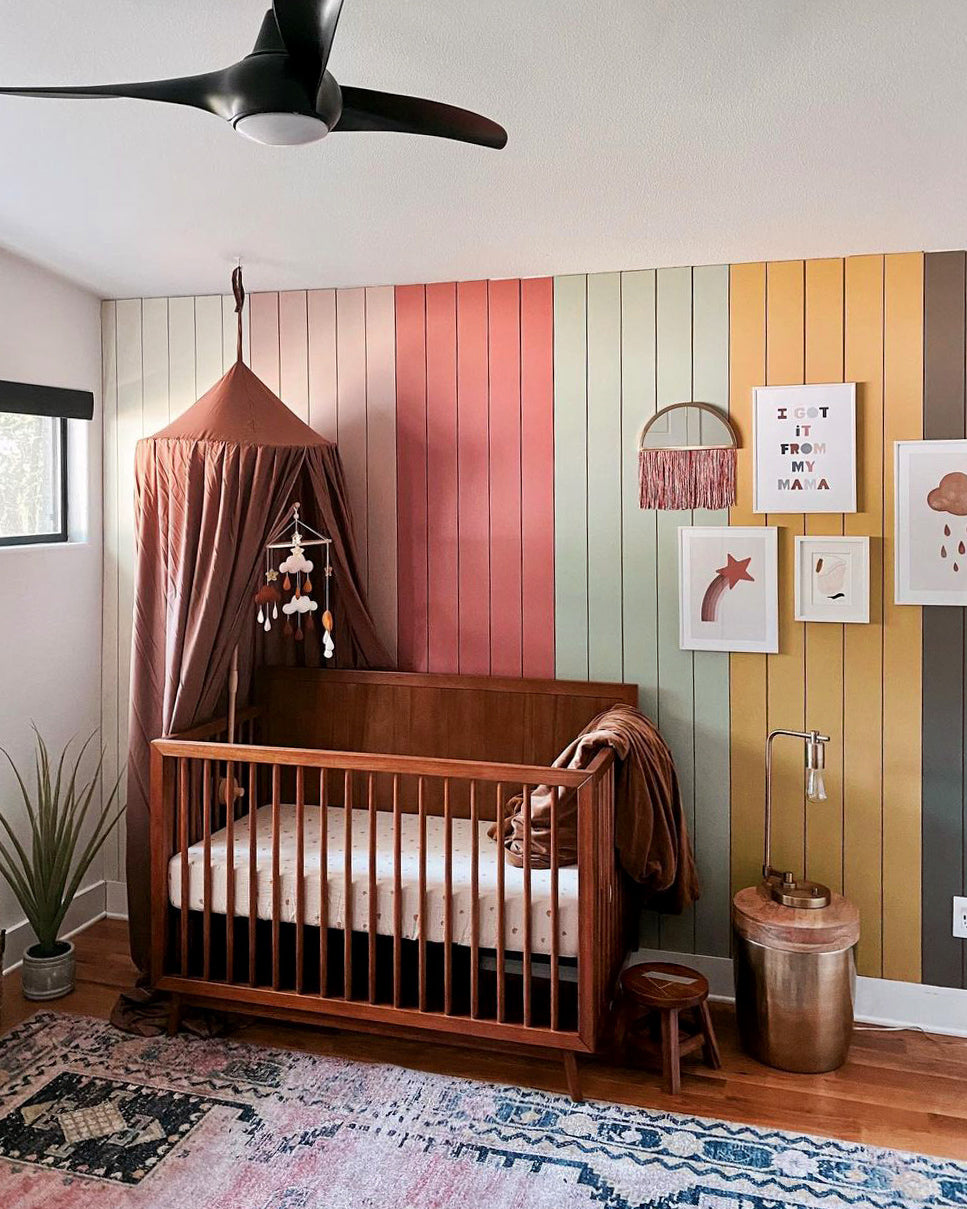This staged and beautifully captured nursery photograph showcases a cozy and vibrant corner of a child's room, perfect for a catalogue. The room features polished honey-colored wooden flooring and simple white ceiling with a ceiling fan that has two blades and a central round light. The focal point is a dark brown wooden crib, set against a vertically paneled wall painted in a palette of pale green, dark pink, light pink, mint, yellow, and brown. Above the crib, there is a brown canopy and a delicate mobile hanging, adding a whimsical touch. The right wall includes a window with black frames that lets in natural light. Beneath the window, there is a decorative pot plant and a patterned rug featuring red, white, and blue hues. Additionally, the wall is adorned with four framed posters and a charming tassel-adorned rainbow. A small bedside table with a lamp and a stool completes the cozy arrangement.